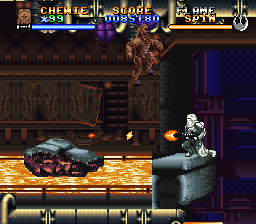In this screen capture from a Star Wars video game, we see a high-intensity showdown between the iconic character Chewbacca and a formidable Stormtrooper. Chewbacca, commonly known as "Chewie," is prominently featured in the scene, with his life meter displayed below him reading 99. The screen also indicates that players have access to a special move called "flame spin." Chewbacca is depicted in mid-action, seemingly leaping from a vehicle that appears to be traversing a river of lava or flames. The Stormtrooper is actively engaging Chewbacca, emitting a stream of fire towards him. Despite the dark and somewhat ambiguous details in the animation, the dynamic and fiery clash between Chewbacca and the Stormtrooper captures the thrilling essence of the Star Wars-themed gameplay.